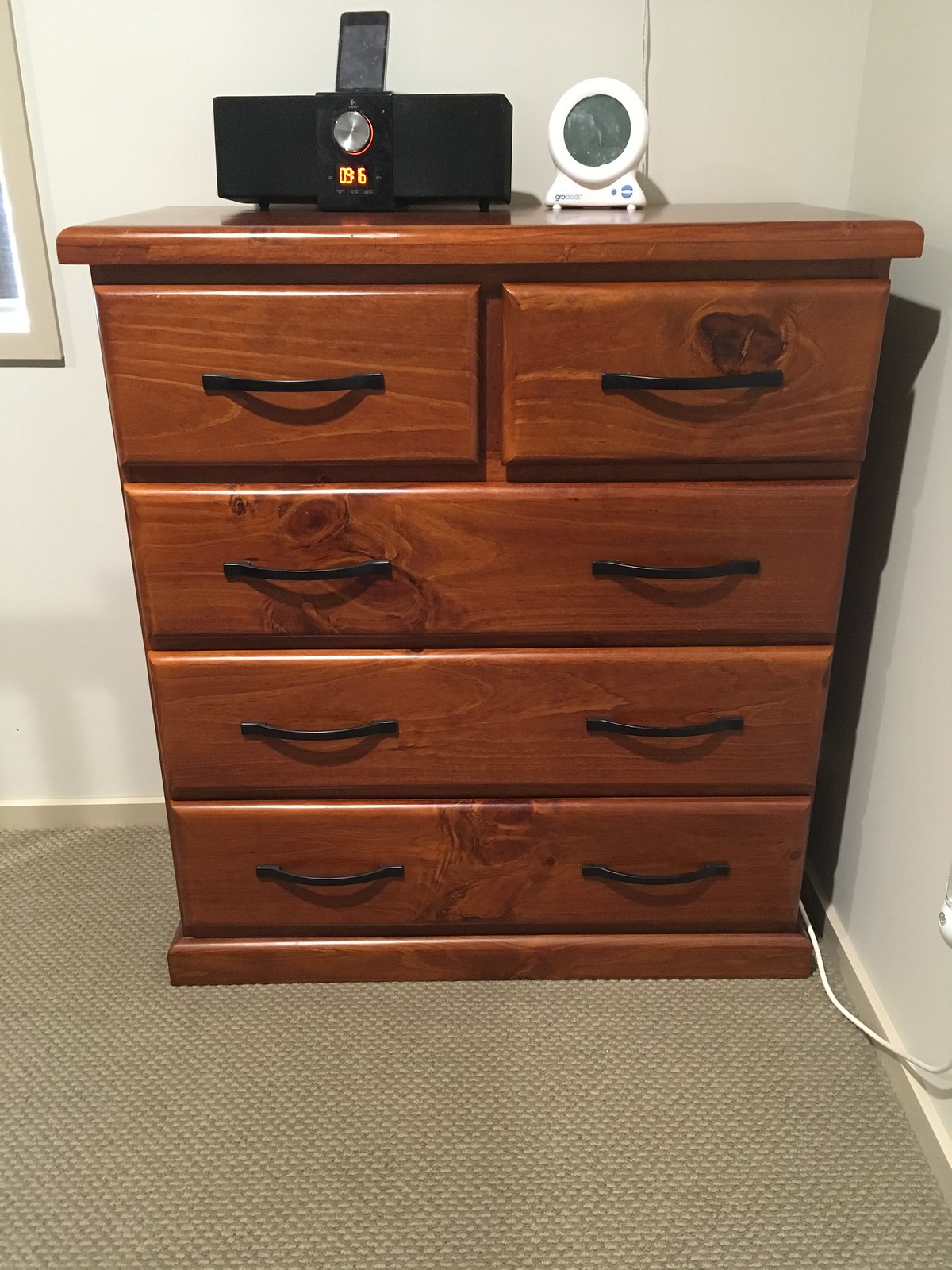This image showcases a chest of drawers, also known as a dresser, situated in the corner of a room with cream-colored walls. The chest is crafted from a reddish-orange wood, characterized by visible knots and a natural finish. It has a total of five drawers: the top section features two smaller drawers that span half the width of the chest, and below these are three larger, full-width drawers, each fitted with black handles.

The room features a light brown or beige patterned carpet, adding a subtle contrast to the darker dresser. In the background, a window pane with a brown frame is visible on the upper left side of the image, along with the edge of a framed picture on the wall. A white coat is draped in the bottom right corner, either on or near the dresser.

On top of the dresser, several electronic devices are displayed: a rectangular black speaker with a silver dial and red text on its display, likely serving as a music system; an iPhone or iPod Touch is connected atop this speaker. To the right of the speaker sits a white circular device, probably another speaker or a clock, characterized by a gray center and a dial at its base. 

Overall, the scene is a blend of warm wood tones and modern electronic elements, set against a soft, neutral backdrop.